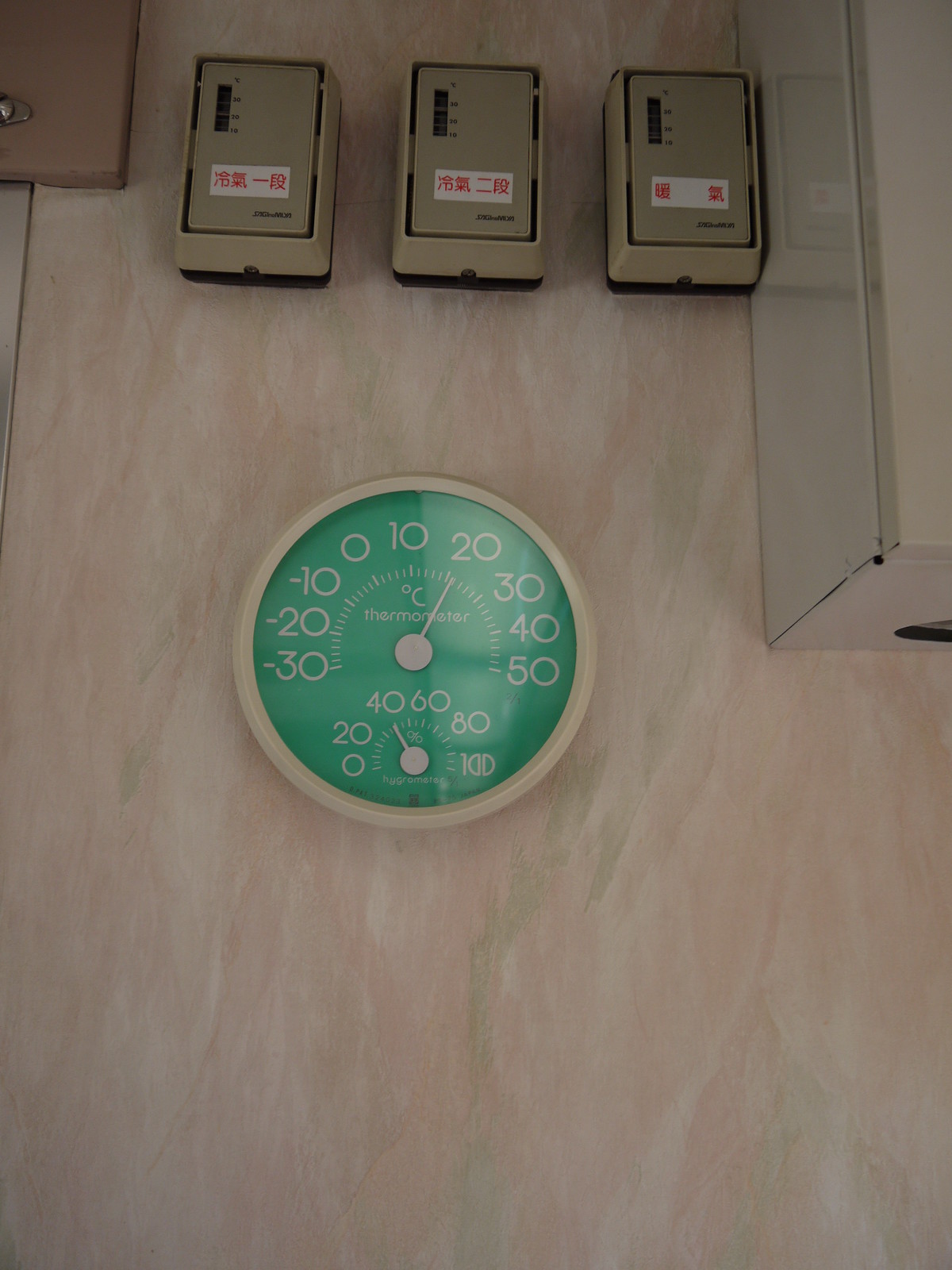A detailed color photo in portrait orientation captures an eclectic array of objects on a surface, which upon closer inspection, appears to be a piece of light-colored unfinished plywood, characterized by its subtle grain. 

In the top right corner and extending halfway down the right edge of the image sits a long, rectangular tan metal box reminiscent of a file drawer or a safe deposit box. The top surface of this box is visible, contributing to its sturdy, industrial appearance.

Spanning the uppermost portion of the photo are three identical, rectangular objects, which closely resemble thermostats. They are two-toned with tan tops and black bottoms and feature white labels adorned with red Chinese or possibly Japanese characters. The first label appears to bear the character for the number one, the second for the number two, while the third is curiously blank in its center. The purpose of these objects is uncertain—potentially plastic containers or even business card holders.

Below them, a round object draws attention. Clock-like in design, this white-framed device is, in fact, a thermometer with a green dial face. It features two measurement dials: the larger top dial ranges from -30 to +50 degrees Celsius, currently indicating 20 degrees. The smaller bottom dial measures humidity, ranging from 0 to 100%, presently reading 40%.

This well-lit, detailed composition combines elements of the mundane and the mysterious, unified by the natural, raw backdrop of unfinished plywood.